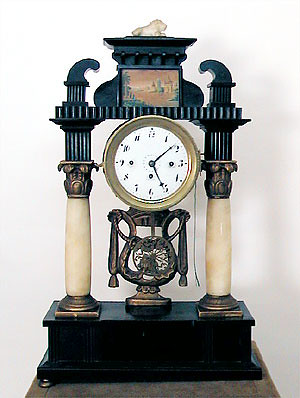This detailed image captures an antique, vintage-looking clock, likely from the 1700s or 1800s. The clock has a black rectangular wooden base that serves as a platform, with four rectangular drawer-like features at the front. Resting on this base are two prominent ivory pillars, each adorned with intricate copper or brass designs at their tops.

The clock itself features a white face with black numbers, ranging from 1 to 12, and minute marks. The black minute and hour hands are clearly visible, and there are three winding holes on the clock face. The central section of the clock includes an ornate brass design, possibly resembling a lyre or similar intricate pattern. 

On top of the structure, there is a smaller black platform with an Asian-inspired style. Crowned at the very top of the clock is a detailed white statue of a lion or tiger, adding to the clock's majestic and classical appearance. The overall design includes brownish and gold details that complement the decorative and stately aesthetic of the timepiece.